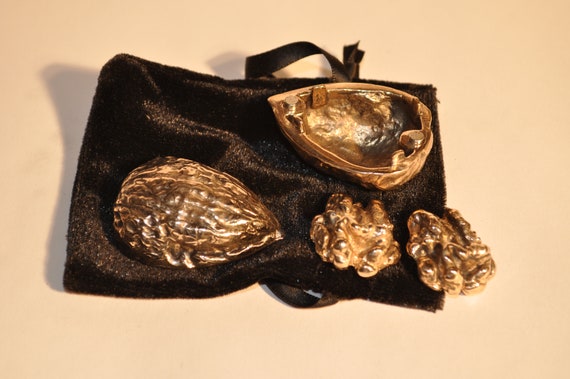The image features two halves of a walnut shell and two pieces of walnut meat, all appearing to be coated in gold. The walnut shell halves are intricately detailed, with one half facing up to reveal its concave interior, showcasing connecting stubs, while the other half is face down, with its convex exterior visible. The pair of walnut meat pieces display a rough texture and uneven surface, also dipped in gold. These items rest on a luxurious black satin drawstring bag, used for gifting, which casts a shadow towards the left side of the image. The bag's opening points to the right, and the scene is set against a light cream-colored background with lighting illuminating from the right.